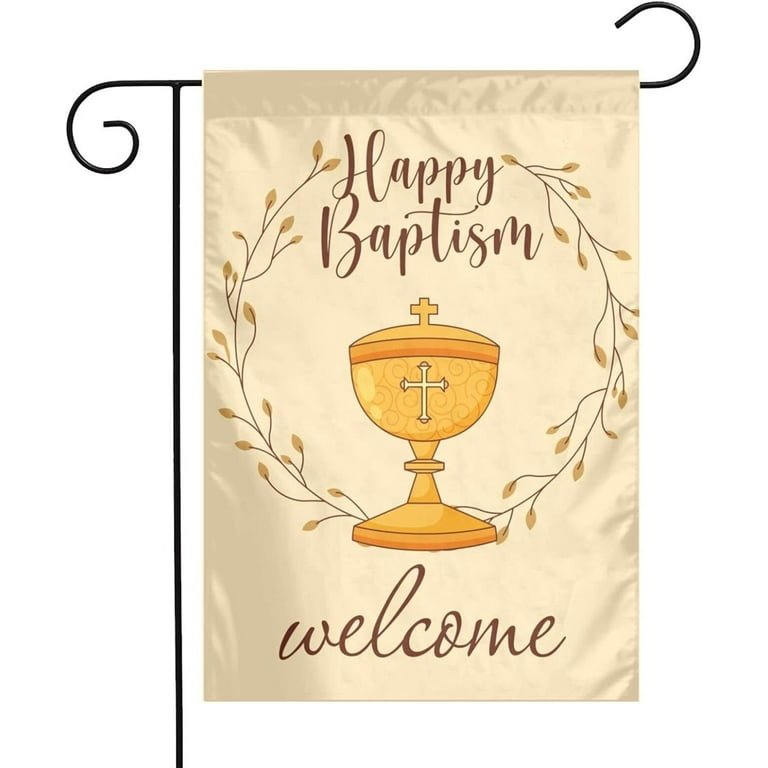This image features a yard decoration against a bright white background, resembling an item you might order online. The centerpiece is a cream-colored, silky fabric banner with decorative elements designed for a baptism event. The banner is attached to a black, ornamental metal pole that can be staked into the ground. The banner features the phrase "Happy Baptism" in a playful cursive script, framed by U-shaped olive vines that evoke the elegance of a Caesar's wreath. Below the text is a depiction of a chalice adorned with a cross on both the lid and the front. At the very bottom, the banner warmly invites with the word "Welcome" in the same cursive script. The lettering throughout is a warm, medium brown, enhancing the overall delicate and welcoming tone of the decoration.